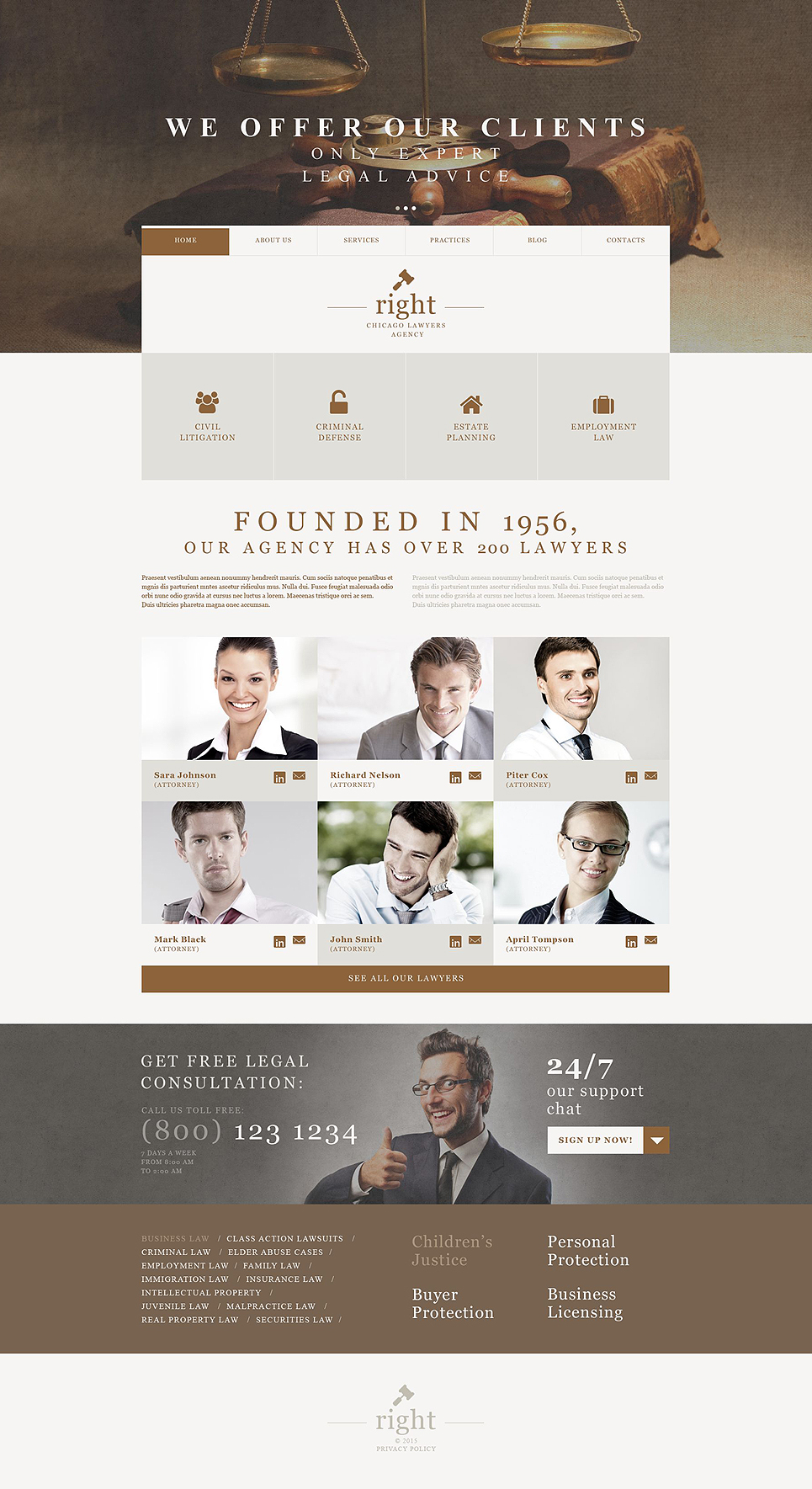Screenshot of Legal Advice Website: 

The website screenshot features a prominent heading at the top that reads, "We Offer Our Clients Only Expert Legal Advice." A graphic of two scales symbolizes the pursuit of justice and underscores the site's legal focus. Below the heading, several navigation buttons provide easy access to different areas of legal expertise, including Civil Litigation, Criminal Defense, Estate Planning, and Employment Law. 

Established in 1956, the agency boasts a robust team of over 200 lawyers. The site includes individual profiles of various attorneys. Among them are Sarah Johnson, Richard Nelson, Peter Cox, Mark Black, John Smith, and April Thompson, all listed as attorneys. Each profile appears to provide specific details about the lawyers' qualifications and areas of specialization.

For potential clients, the website offers a phone number for a free consultation: 1-800-123-1234. Accompanying the contact information is an eye-catching image of a man in a suit, giving a thumbs up and smiling broadly. His exaggeratedly large eyes and enthusiastic expression aim to project approachability and confidence.

Additionally, the website highlights 24/7 chat support, indicating round-the-clock assistance for visitors in need of immediate legal advice.